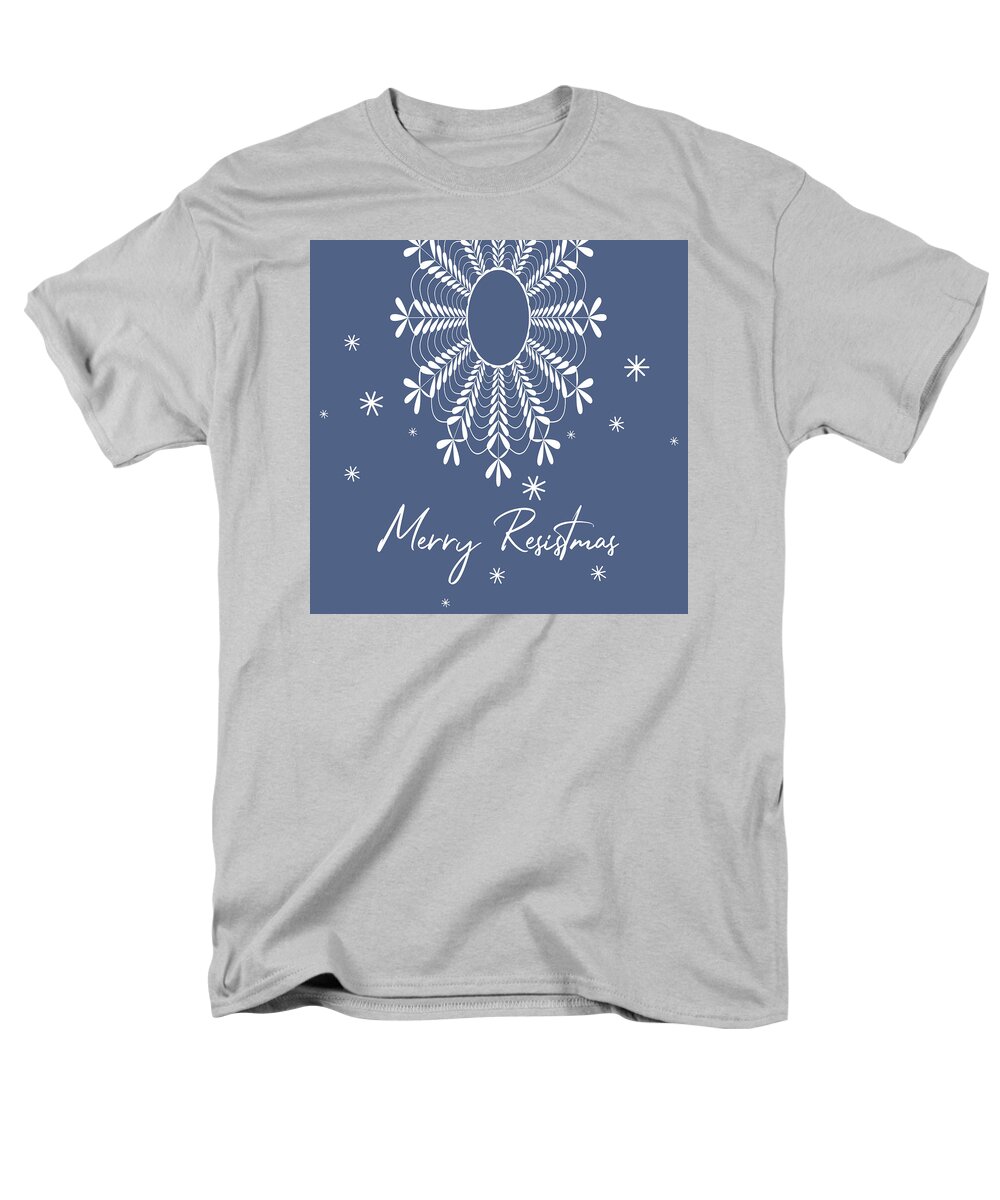The image depicts a heather gray, short-sleeved t-shirt laying on a white background. The t-shirt appears to be a regular fit with no visible label. On the chest of the t-shirt, there is a large slate blue square which occupies about half of the shirt's front. Inside this square, the phrase "Merry Resistmas" is printed in white cursive text. The center of the square features a prominent, intricate white snowflake design surrounded by smaller white snowflakes scattered towards the sides and bottom. There is also a distinct blue circular element within the central snowflake that connects to the surrounding pattern, contributing to its unique web-like appearance.